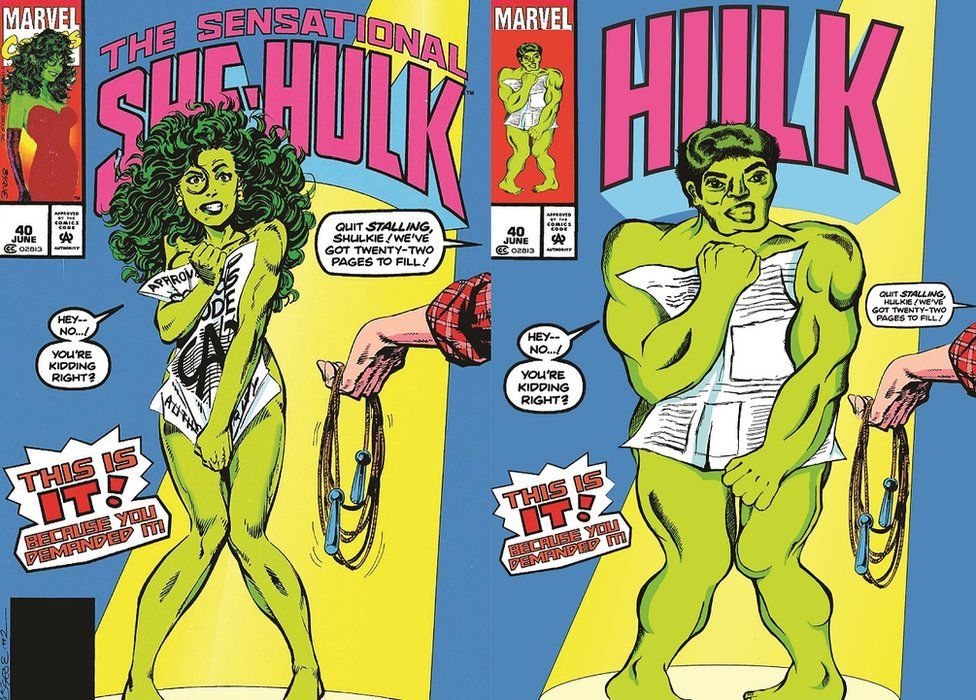The photograph depicts two Marvel comic book covers side by side. On the left cover, titled "The Sensational She-Hulk" in bold, pink text at the top, a green-skinned woman with dark green hair is featured holding a newspaper in front of her naked body. A speech bubble from her reads, "Hey, no, you’re kidding, right?" Below this, in red text with a white outline, it states, "This is it! Because you demanded it." 

The right cover mirrors the left, showing a male Hulk with a broad, muscular frame, also holding a newspaper to cover his nudity. He shares the same speech bubble, exclaiming, "Hey, no, you’re kidding, right?" Above him, the title "Hulk" is displayed in three-dimensional pink letters.

In both covers, a hand clad in a rolled-up red checkered shirt extends from the right edge, holding a rope with two blue handles. A speech bubble from off-frame commands, "Quit stalling, Shulky/Hulky. We’ve got 22 pages to fill." Each background features a distinctive blue and yellow color scheme, and both titles prominently display the Marvel logo.